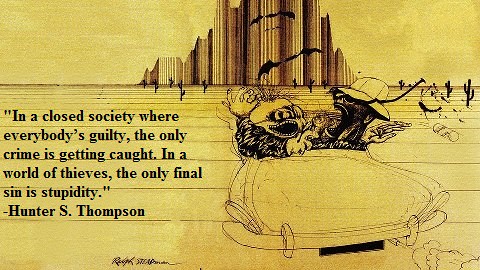The image appears to be a postcard with a dirty yellow background, featuring an intricate black ink or pencil drawing. Dominating the left side, the caption reads, "In a closed society where everybody's guilty, the only crime is getting caught. In a world of thieves, the only final sin is stupidity." Attributed to Hunter S. Thompson, this quote is followed by an out-of-focus signature that begins with "Ralph."

In the center of the image, towering brown columns, possibly representing a futuristic cityscape or a series of cliffs, rise into the sky. The bottom of the image showcases a peculiar convertible car, emitting exhaust from its tailpipe on the lower right. This vehicle is populated by three bizarre characters with caricatured, almost monstrous features—one sporting a white hat and another with an open mouth revealing teeth, adding to their goblin-like appearance.

The foreground is dotted with black cacti, with several small ones protruding from the ground on the right and some scattered above the car. Yellow lines stretch across the bottom from left to right. The characters in the car seem to be interacted animatedly, contributing to the chaotic, yet comedic nature of the scene. The overall composition marries elements of whimsy and surrealism, with a desert-like atmosphere punctuated by cacti and the odd car journey seemingly headed towards the mysterious tall structures in the background.